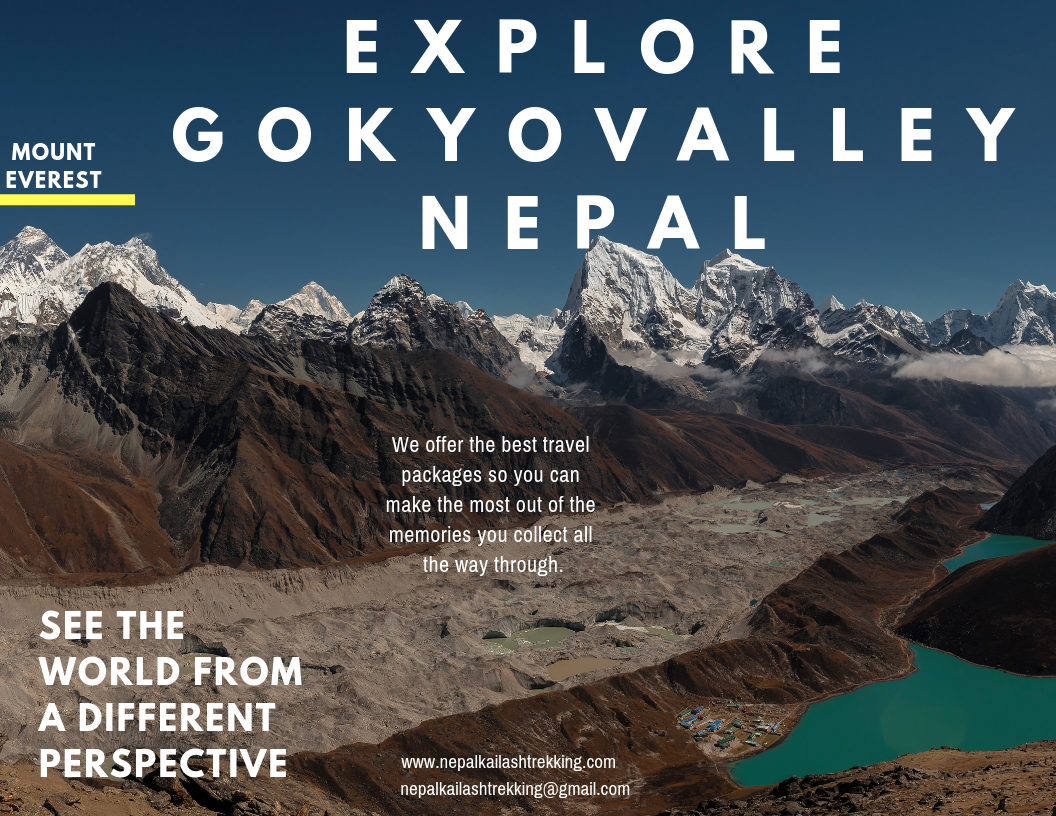Promotional image for visiting Nepal's Gokyo Valley, featuring striking mountainous terrain and remarkable geological features. The background showcases a majestic mountain range, including the iconic Mount Everest marked by yellow underlining and situated on the left side. The rocky features transition from brown mountains in the forefront to snow-capped gray peaks in the distance. Nestled in the lower part of the image is a tiny village by a greenish-blue lake, emphasizing the vast elevation. Additional bodies of water, including teal-colored lakes, are scattered throughout the valley. Bold white text overlays the blue sky, promoting, "Explore Gokyo Valley in Gokyo Valley, Nepal," followed by a message stating, "We offer the best travel packages so you can make the most out of the memories you collect all the way through." Another line of text at the bottom left articulates, "See the world from a different perspective." For more information, visit www.NepalKailashTrekking.com or contact NepalKailashTrekking@gmail.com.